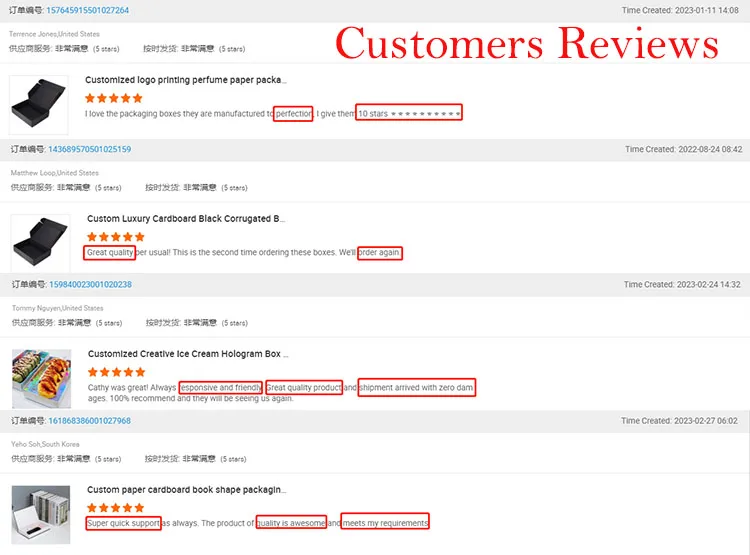The image showcases a series of customer reviews for various customized packaging products, with key details and highlights as follows:

1. **Terrence Jones, United States**  
   - **Timestamp**: 2023-01-11 at 14:08  
   - **Product**: Customized Logo Printing Perfume Paper Packs  
   - **Rating**: Five Orange Stars  
   - **Review**: "I love the packaging boxes, they are manufactured to perfection. I give them ten stars."  
   - **Highlights**: "Perfection" and "ten stars" are emphasized.

2. **Matthew Luke, United States**  
   - **Product**: Custom Luxury Card Box, Black Corrugated  
   - **Rating**: Five Orange Stars  
   - **Review**: "Great quality per usual. This is the second time ordering these boxes, we'll order again."  
   - **Highlights**: "Great quality" and "order again" are marked in red with a box around them.

3. **Tommy Nugent, United States**  
   - **Product**: Customized Creative Ice Cream Hologram Box  
   - **Rating**: Five Orange Stars  
   - **Review**: "Kathy was great, always responsive and friendly. Great quality products, and shipment arrived with zero damages. 100% recommend, and they will be seeing us again."  
   - **Highlights**: "Responsive and friendly," "great quality products," and "shipment arrived with zero damage" are boxed in red.

4. **Yoho, South Korea**  
   - **Timestamp**: 2023-02-27 at 06:02  
   - **Product**: Custom Paper Cardboard Book Shape Packaging  
   - **Rating**: Five Orange Stars  
   - **Review**: "Super quick support, as always. The product of quality is awesome and meets my requirements."  
   - **Highlights**: "Super quick support," "quality is awesome," and "meets my requirements" are boxed in red.

Across the top right, above the reviews, is the text "Customer Reviews" in big red letters. Each review includes a mix of English text and "oriental" (presumably East Asian) characters, indicating a diverse range of customers. Detailed timestamps and product descriptions are noted, ensuring clarity and context for each feedback entry.